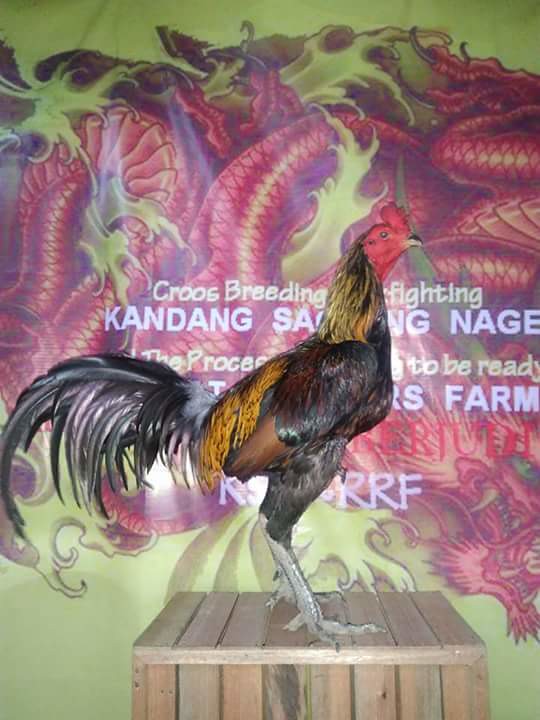In this rectangular image, which is taller than it is wide, a vibrant rooster stands prominently on a light wooden crate at the bottom center. The rooster, facing to the right, exhibits a striking array of colors: a red comb and face, a brown and black feathered neck, dark brown and black wings, a yellowish-orange back, and oily black tail feathers. Its feet are gray and scaly. Above and behind the rooster, the background transitions from a darker green at the top to a faded yellow-green at the bottom. A large red-scaled dragon with long black curled claws and intricate details, reminiscent of the traditional Chinese style, weaves through the background, creating a dynamic scene with splashes of green appearing like water around its body. In the upper right-hand corner, part of the dragon's hind leg and foot are visible, while in the lower right-hand corner, the dragon's head with long singular fangs and whiskers can be seen. Scrawled across the background in white letters are partially obscured words that read "Cruz Breeding Fighting, Kandang, and NAGE. The word "farm" is also visible, though some letters are hidden behind the large, colorful rooster.